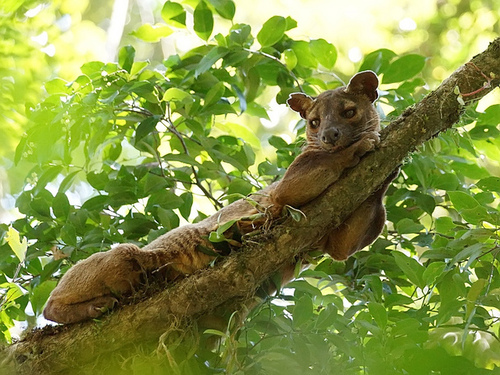The image depicts an outdoor scene bathed in sunlight, with green leaves filling the background and the foreground, creating a smudged, almost fading effect. In the center, a long, limber creature with dark eyes, a rounded nose, and whiskers is draped across a brown, moss-coated branch. The animal has a rusty brown coat, pointed ears with pieces missing, and pronounced claws on its thick legs. It possesses a cat-like body but has distinguishing features reminiscent of a bat, particularly in its facial structure. Stripes are visible on its underbelly, and it appears to be intently gazing at something below, adding an air of mystery to its identity. The leaves around it blur together, with light filtering through, enhancing the dreamy, surreal atmosphere of the scene.